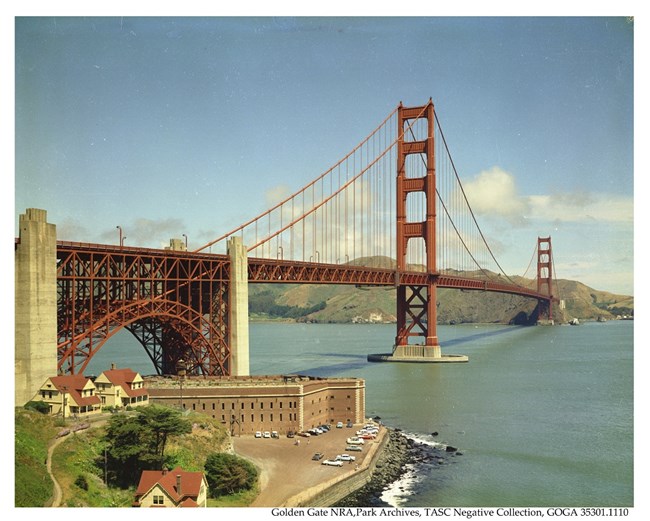This vibrant, daytime photograph captures the iconic Golden Gate Bridge in San Francisco spanning diagonally from the left middle to the right middle of the frame. The bridge, with its distinctive rusty-orange hue, stretches majestically over the calm waters of the San Francisco Bay. In the foreground, there is a long building situated in the lower left corner with a parking lot bustling with parked cars. Surrounding the building, a couple of houses with orange roofs are visible, connected by a winding path lined with grass and some trees. The backdrop features mountains shrouded in white clouds against a clear blue sky. Additional details include the surrounding islands and part of the shoreline adorned with smooth waves lapping gently. Notably, the photo is marked with the inscription "Golden Gate NRA Park Archives TASC Negative Collection GOGA 35301.1110."